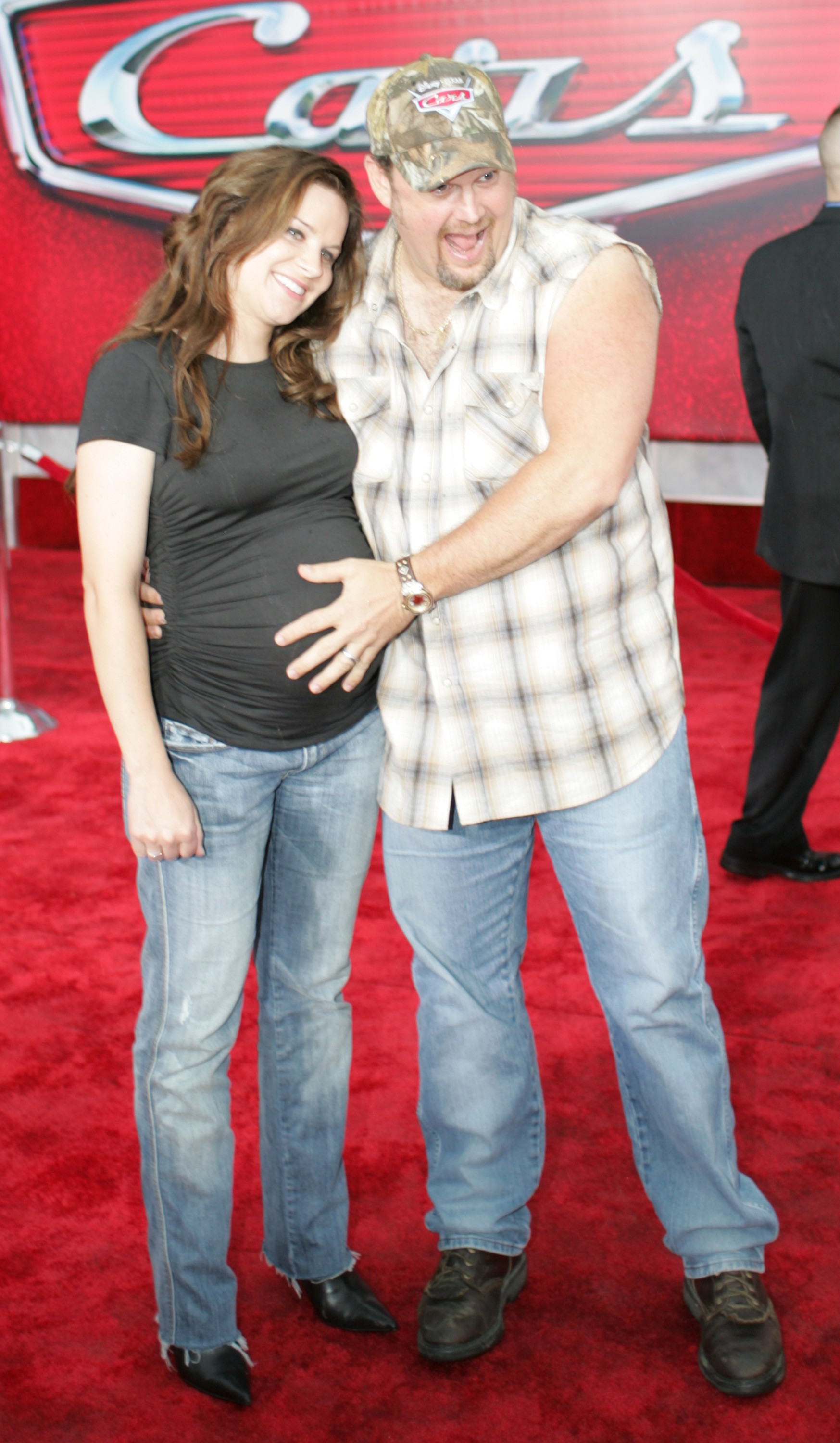In this vibrant photograph taken at what appears to be the "Cars" movie premiere, two people joyously pose on a striking red carpet. To the left stands a woman in her 30s, with loose wavy brown hair cascading just past her shoulders. She wears a black short-sleeved shirt that stretches over her noticeably enlarged belly and blue jeans with frayed hems at the ankles, complemented by pointed black leather high heels. Her right arm hangs casually by her side, her hand loosely balled into a fist. She tilts her head affectionately towards the man beside her, smiling brightly.

Next to her is a muscular Caucasian man, identified as Larry the Cable Guy. He is dressed in a white sleeveless button-up plaid shirt with the top two buttons undone, blue jeans, and brown boots with light brown laces. His shirt's sleeves have been torn off, and his left arm wraps gently around the woman's back, with his left hand resting protectively on her waist. His right hand is cradling her belly. Larry sports a camouflage green foliage-pattern hat that reads "CARS" in a rectangular field. He also wears a gold watch and has a connected mustache and goatee. Both appear content and excited.

The backdrop features a prominent "CARS" logo in a vintage 1950s-style cursive, bordered with metallic detailing, evoking a sense of nostalgic charm. The red background behind them is marked by subtle variations in shade, adding depth to the image. Off to the right, partially cut off, is another man in a black suit, facing away from the camera and walking out of the frame, adding an air of curiosity to the setting. The couple stands amidst a sea of red hints and metallic elements, perfectly framing this joyous and celebratory moment.